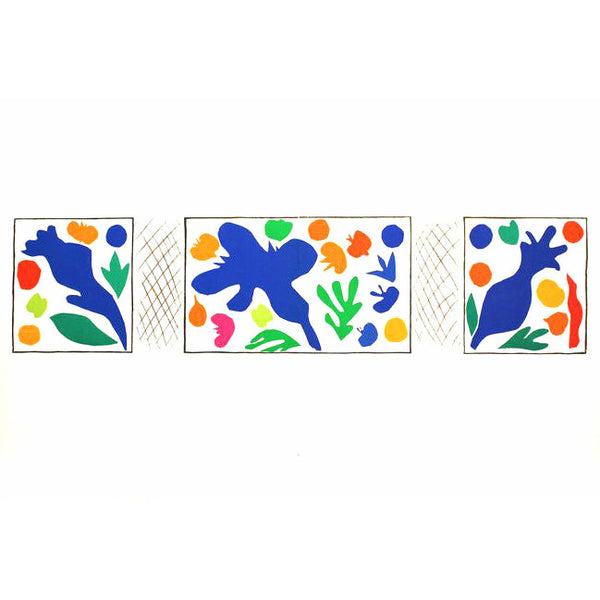The image depicts a triptych artwork, meticulously framed in thin black frames. The composition features a central rectangular piece flanked by two smaller square side pieces, all set against a solid white background. Each of the three panels showcases an array of abstract shapes richly colored in blue, lime green, yellow, orange, pink, and green. A dominating design element is a complex, large abstract shape in dark blue present in each of the panels, surrounded by splotches and circular patterns in vibrant hues of orange, green, and blue. These shapes are interspersed with leaf-like designs in green. Intensity and repetition of orange splotches are noticeable across all panels, providing a sense of cohesion and flow. The overall design is further accentuated by a cross-hatched pattern that connects the side pieces to the central artwork, enhancing the unified yet distinct presentation of the triptych.